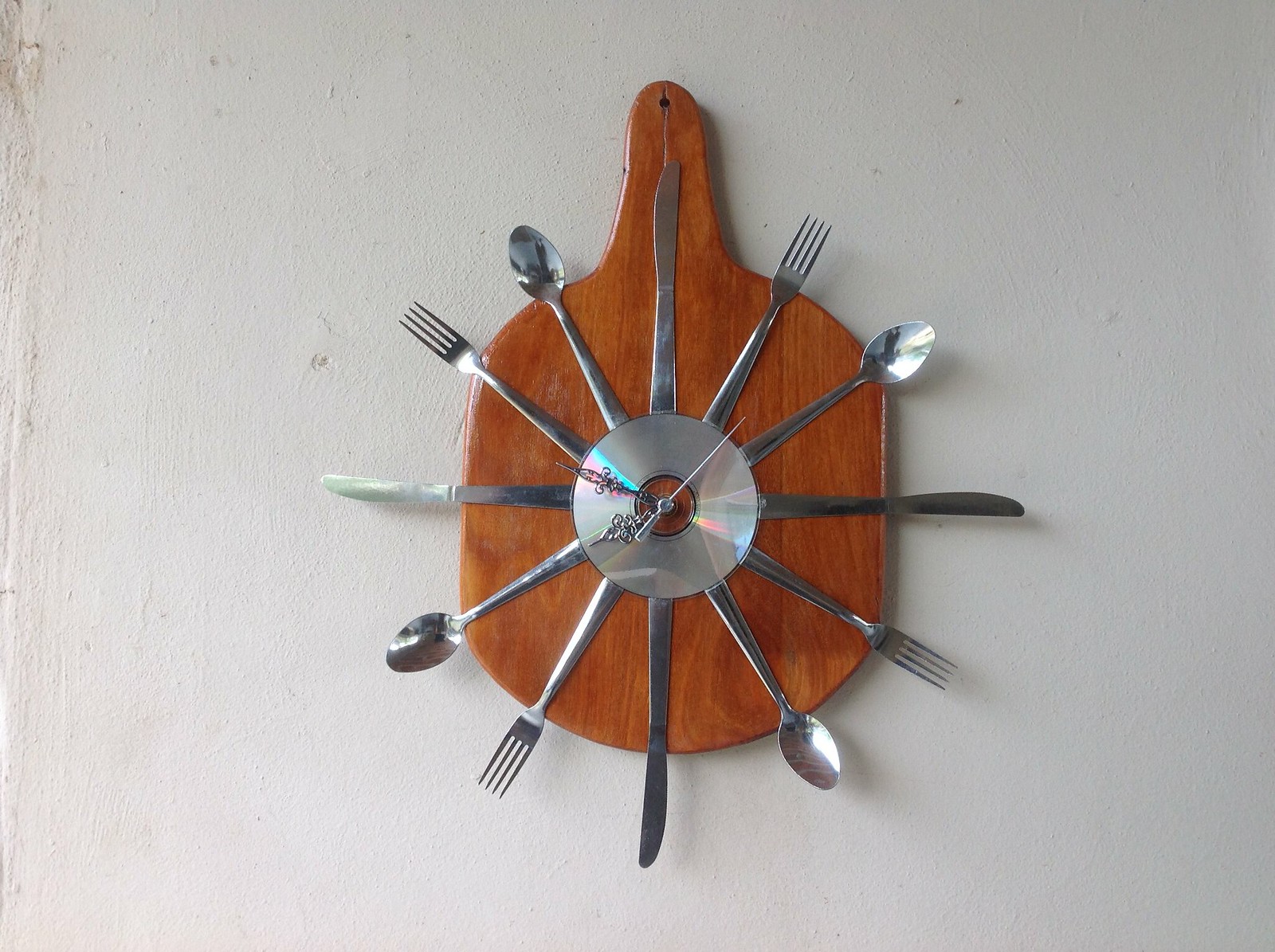This color photograph captures a unique wall-mounted clock crafted from a medium brown, beautifully polished wooden chopping board shaped like a paddle or ping pong bat, with a handle at the top. The clock is mounted on a light gray, possibly white, wall. At its center is a CD, serving as the clock face, and the clock hands—a slender sweep-second hand, delicate minute hand, and hour hand—are elegant with silver filigree patterns. Instead of numbers, silver kitchen utensils represent the hours: starting from the top, a knife marks the 12 o'clock, a fork at 1 o'clock, and a spoon at 2 o'clock. This pattern of knife, fork, spoon then repeats around the face of the clock: with knives at 3, 6, and 9 o'clock, forks at 4, 7, and 10 o'clock, spoons at 5, 8, and 11 o'clock. The second hand points between 1 and 2 (between the fork and spoon), the hour hand points at 8 (a spoon), and the minute hand points between 9 and 10 (between the fork and knife).